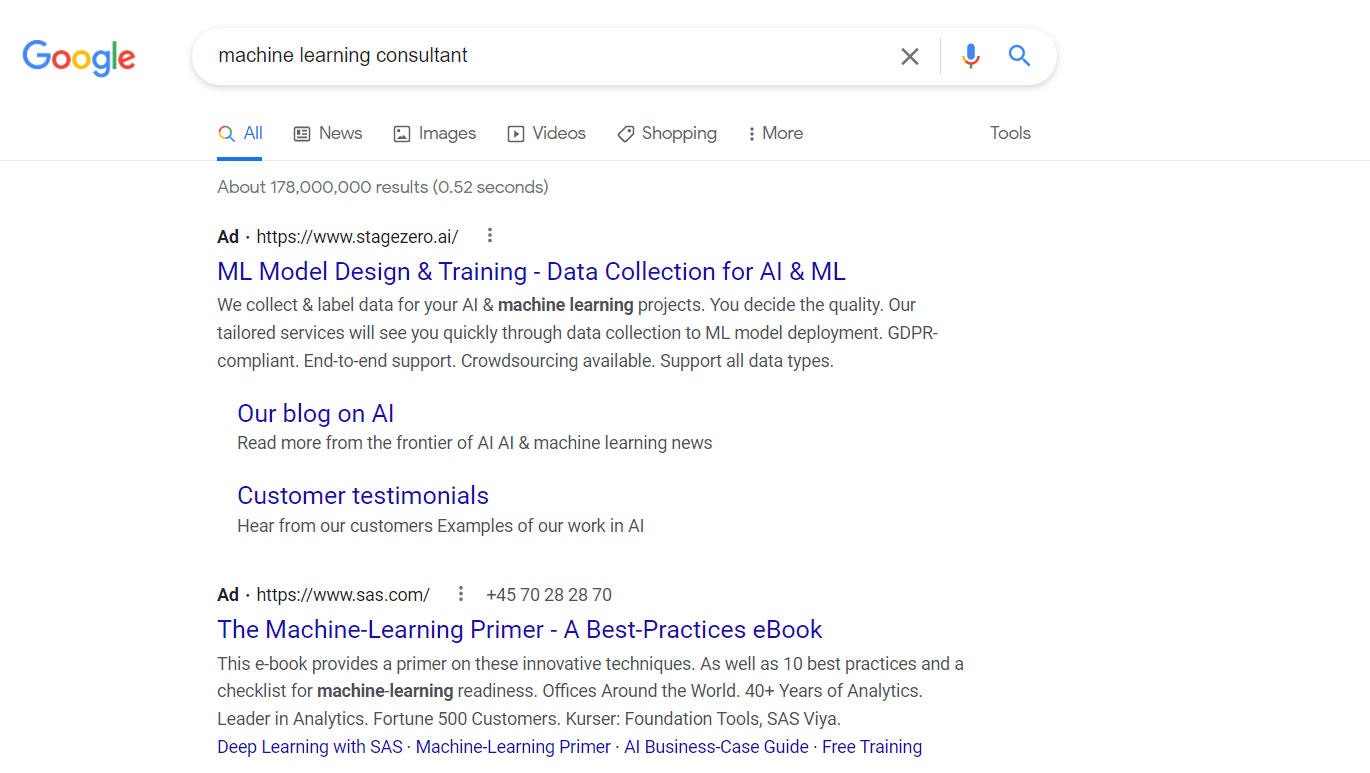This is a detailed screenshot of a Google search results page. On the left, the iconic Google logo is prominently displayed. Centered in the page is the search box containing the phrase "machine learning consultant," flanked by an 'X' for clearing the text, a microphone icon for voice input, and a magnifying glass for initiating the search. Just beneath the search box are several category filters including 'All,' 'News,' 'Images,' 'Videos,' 'Shopping,' and 'More,' with a 'Tools' option on the far right.

The search results reveal approximately 178,100,000 results generated in 0.52 seconds. The topmost result is a sponsored ad, detailing a service for ML model design and training data collection for AI and machine learning projects. The ad emphasizes high-quality, tailored services that ensure quick data collection to ML model deployment. It highlights GDPR compliance, crowdsourcing support, and compatibility with all data types. A clickable link in blue text reads, "Our Blog on AI," leading to further insights and updates on AI and machine learning developments. Beneath this link, the text "Read more from the frontier of AI" is displayed in a gray font, encouraging users to delve deeper into AI and machine learning news.

Following this is another clickable link titled, "Customer Testimonials," inviting users to hear about customer experiences and review examples of the company's previous AI work. Positioned below the testimonials is another ad, introducing "The Machine Learning Primer — A Best Practices Ebook." This resource offers a primer on innovative techniques, detailing 10 best practices and a checklist for machine learning readiness. Additional text mentions the company's global offices, over 40 years of analytics leadership, and a clientele of Fortune 500 customers. The ad concludes with educational offerings, such as "Deep Learning with SAS" and "AI Business Class Guide — Free Training," all presented in blue text for easy navigation.